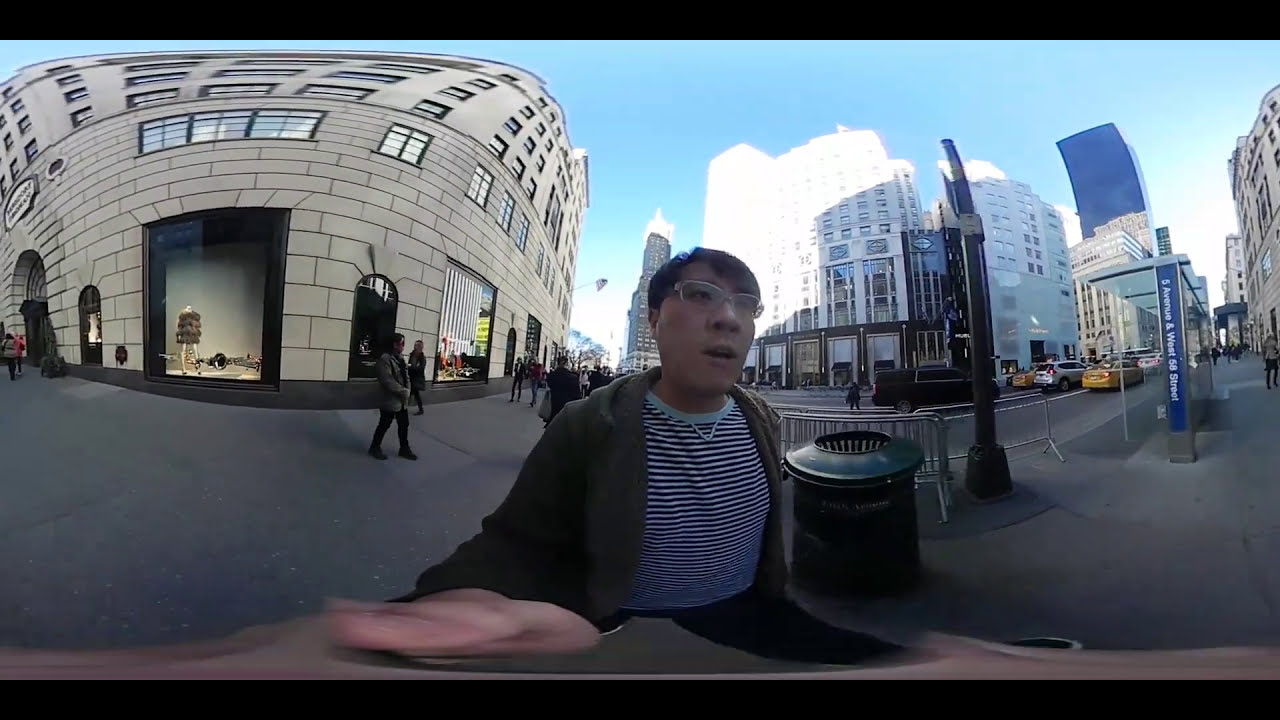In this cityscape image, an Asian man with dark hair and whitish glasses is prominently featured in the center. He appears to be taking a selfie or recording himself with a camera, highlighted by his hand visible holding the device. He is dressed in a blue and white horizontally striped shirt underneath a gray jacket, paired with black pants. The bustling urban environment around him includes various large buildings, primarily white and gray with some tan and beige structures, featuring large windows and a mix of architectural styles. 

Behind him, pedestrians populate the gray sidewalks, moving past store entrances with large display windows, one of which features a mannequin clad in a fur coat or dress. There are also people waiting by a blue bus stop with a small roof. Cars and taxis navigate the city streets, adding to the dynamic scene. Additionally, a garbage can and silver barriers are visible close to the man, enhancing the typical city atmosphere. The sky above is clear and blue, contributing to the vibrant and lively downtown setting in which he seems to be leisurely exploring.